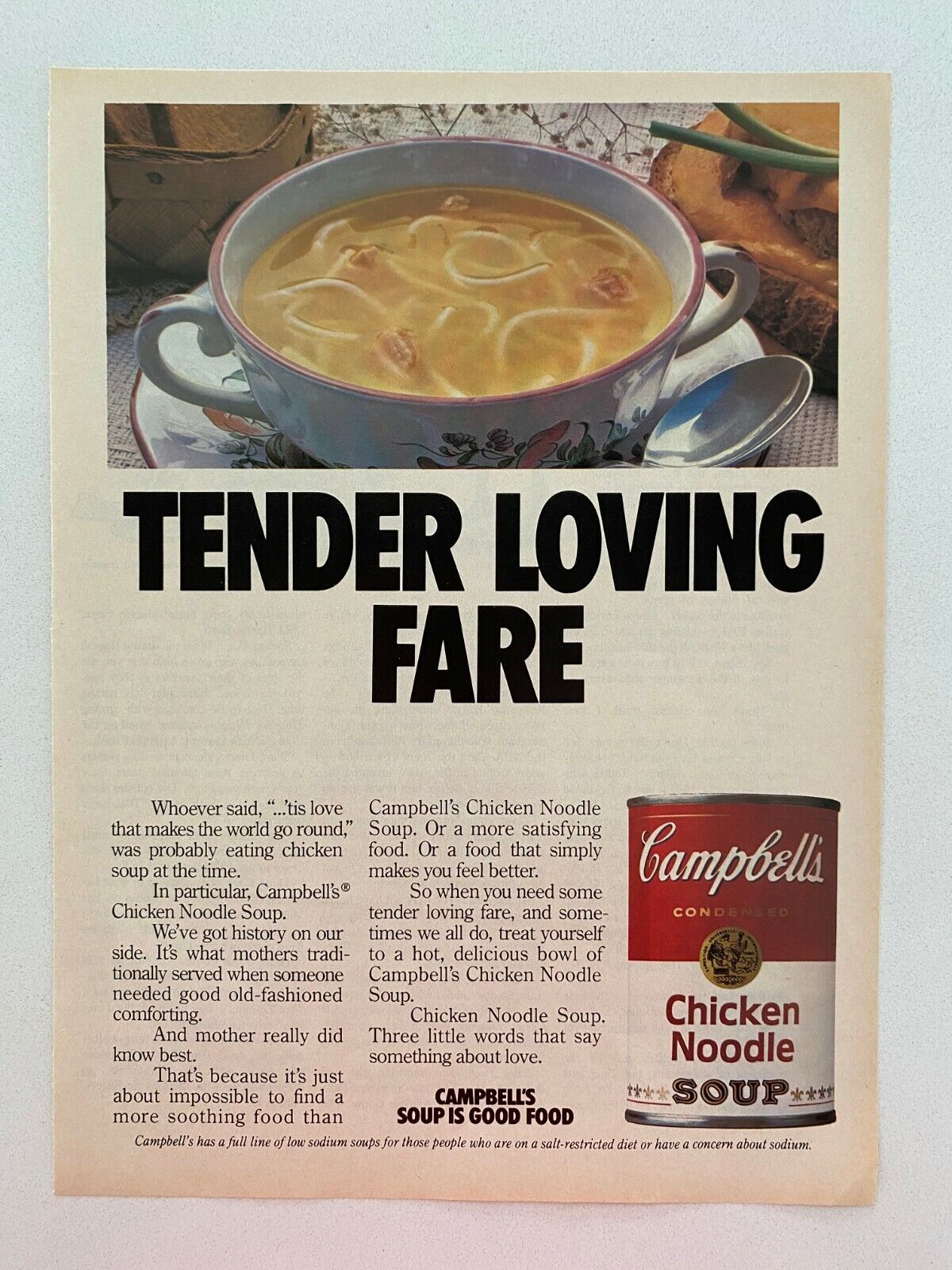This image is a detailed magazine advertisement for Campbell's Chicken Noodle Soup. The ad features a beautifully set scene with a decorative white bowl with floral designs, filled with noodles and accompanied by a spoon, placed on a saucer at the top of the page. The central text boldly reads "TENDER, LOVING, FAIR" in black capital letters, emphasizing the comfort and care associated with the product. Below this, an elaborative description highlights the nostalgic and soothing qualities of Campbell's chicken noodle soup, noting its historical association with comfort and care. The ad mentions phrases like "whoever said love makes the world go round was probably eating chicken soup at the time" and "mother really did know best," reinforcing the comforting nostalgia of the soup. At the bottom right corner, a red and white Campbell's Chicken Noodle Soup can is prominently displayed, underscoring the brand. The background of the page is beige, contrasting with the white surface on which the magazine is placed. Additional text at the bottom of the page declares in bold letters "CAMPBELL'S SOUP IS GOOD FOOD," further anchoring the product's identity. Colors in the ad include black, gold, green, red, silver, and beige, contributing to its visual appeal. The overall style of the advertisement is classic and comforting, aligning perfectly with the product being promoted.